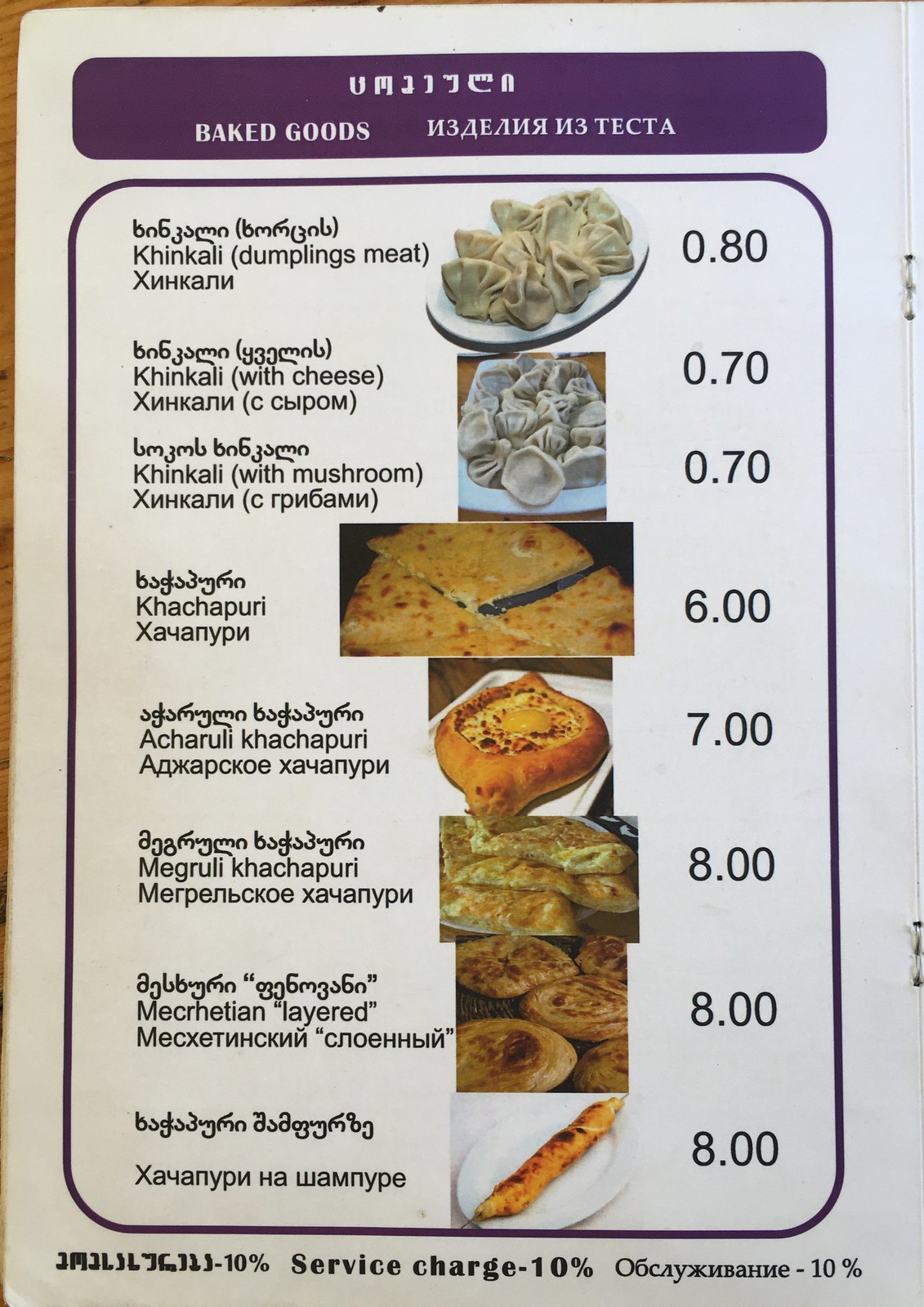This photograph captures a detailed page from a menu, set against a white background. At the top center of the page, there is a purple rectangle with rounded edges. Inside this rectangle, centered at the top, is a row of Arabic characters. Below these characters, slightly to the left, is the text "BAKED GOODS" in white, all-caps letters, and to the right of this, the Arabic translation is also provided. 

Underneath the purple rectangle, a large, black-outlined square with rounded edges features prominently. Inside this square, at the top, there are more Arabic characters written in black. Beneath these characters, the name of the dish is given in alphabetic text. To the right of this description, there is a white oval plate holding several dumplings, with the price listed nearby.

Following this initial description, the menu continues with a total of seven items, each aligned vertically:

1. The first item, described above, features dumplings on a white oval plate with both Arabic characters and translations.
2. The second item, to the right of its description in black text, displays what seems to be white ravioli on a blue round plate.
3. The third item shows pita or flatbread cut into triangles, characterized by an orange hue with brown spots.
4. The fourth item presents a round baked bread with a hollowed-out center filled with an unknown ingredient.
5. The fifth item features white and tan-colored rolls.
6. The sixth item is a circular Danish pastry, light brown in color with a darker center.
7. The final item on the page is an image of golden brown French bread.

Each item is intricately detailed, making the menu both visually appealing and informative.